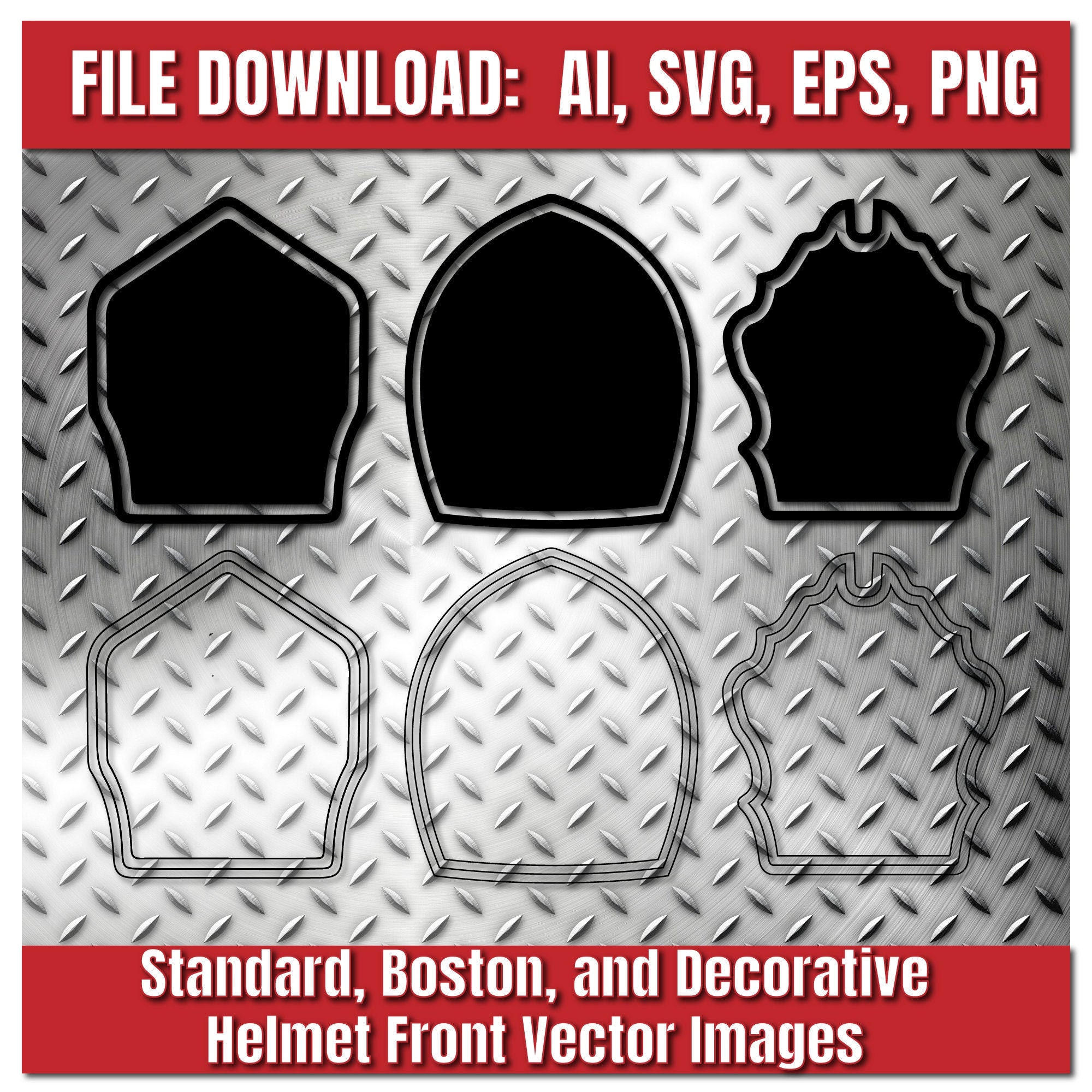The image is a vertical-rectangular advertisement for software, featuring a piece of metal with rivet-like indentations serving as the background. The design is divided into three distinct sections: 

- At the top, there is a red banner with white text that reads "File Download AI, SVG, EPS, PNG."

- In the middle section, six "Helmet Front Vector Images" are displayed in two rows. The top row features three distinct black, filled-in and bordered images, while the bottom row shows the same three images in a more translucent, unfilled style, resembling sketches on the metallic background.

- At the bottom, another red banner with smaller white text reads "Standard Boston and Decorative Helmet Front Vector Images." 

The entire backdrop shows a grayish hue with a hinted grid pattern, adding a textured look to the advertisement.